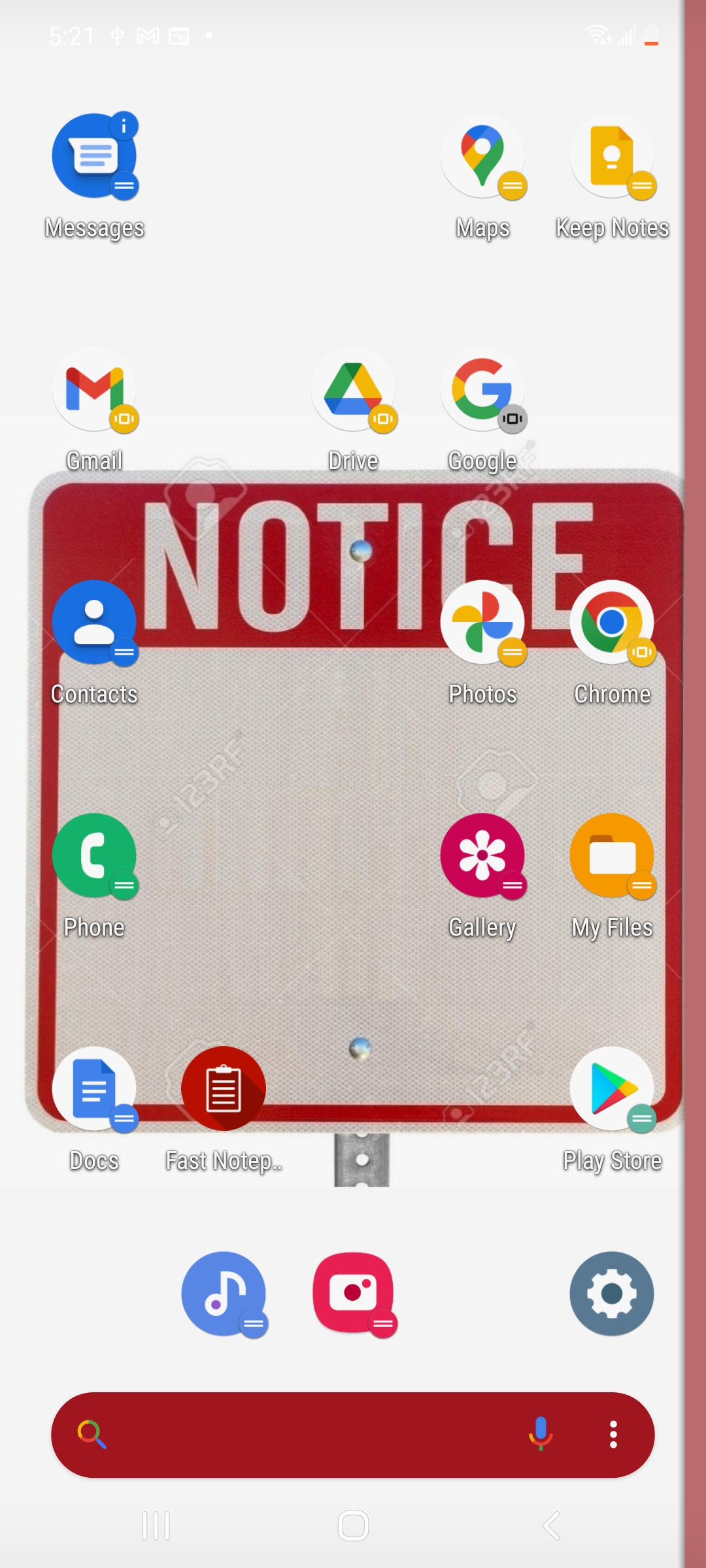This image is a screenshot of an Android phone's home screen, displaying a somewhat disorganized array of app icons against a white background. Among the icons scattered across the screen are commonly used apps such as Gmail, Google Drive, Google Maps, Messages, My Files, Chrome, Google Photos, Phone, Google Docs, and the Play Store, which confirm that this is indeed an Android device. The screen also features the Camera app, a music app, and the Settings button. Prominently displayed at the top is a red 'Notice' label, beneath which lies a large white square devoid of any text. At the very bottom of the screen, a search field is visible. Additionally, there is an indication of an unread message, though the exact number of unread emails is not discernable from the screenshot.